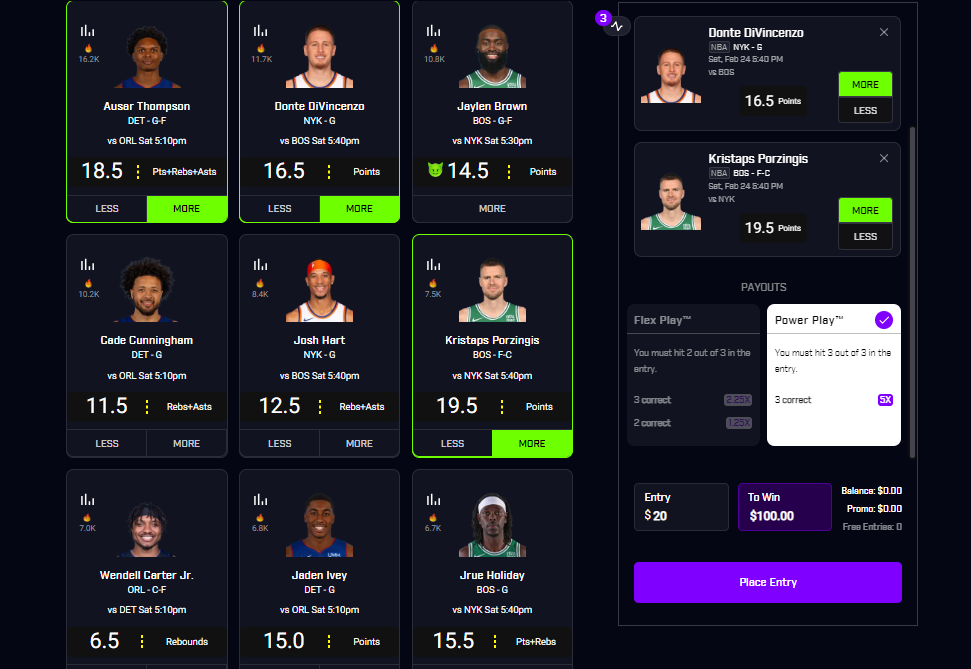The image depicts a sports ranking or online betting website with a sleek, black background. On the left side, the main body of the site features a 3x3 grid of athlete profiles, each consisting of a photograph centered above the player's name and statistical information. Three of these player profiles are highlighted with a green circle, indicating they have been selected. Among the nine visible athletes, there is a mix of two white and seven black sportsmen, suggesting the sport might be basketball.

On the right side of the site, a vertical scroll bar is present, with interactive elements situated along this margin. At the top, two athlete profiles are displayed, each including a profile picture, the player's name, and relevant stats. Adjacent to these profiles is a prominent neon green button labeled "More." Below these, a section titled "Playlists" can be seen, followed by another segment named "Flex Play," which includes additional details. 

Further down, a white block marked "Power Play" is highlighted, indicating it is currently selected. A note within this section suggests that three out of three entries must be fulfilled. At the very bottom of the right-hand side, next to the scroll bar, there's text indicating that an entry fee of $20 could yield a potential win of $100, alongside a button to "Place Entry," hinting at the site's betting functionality.